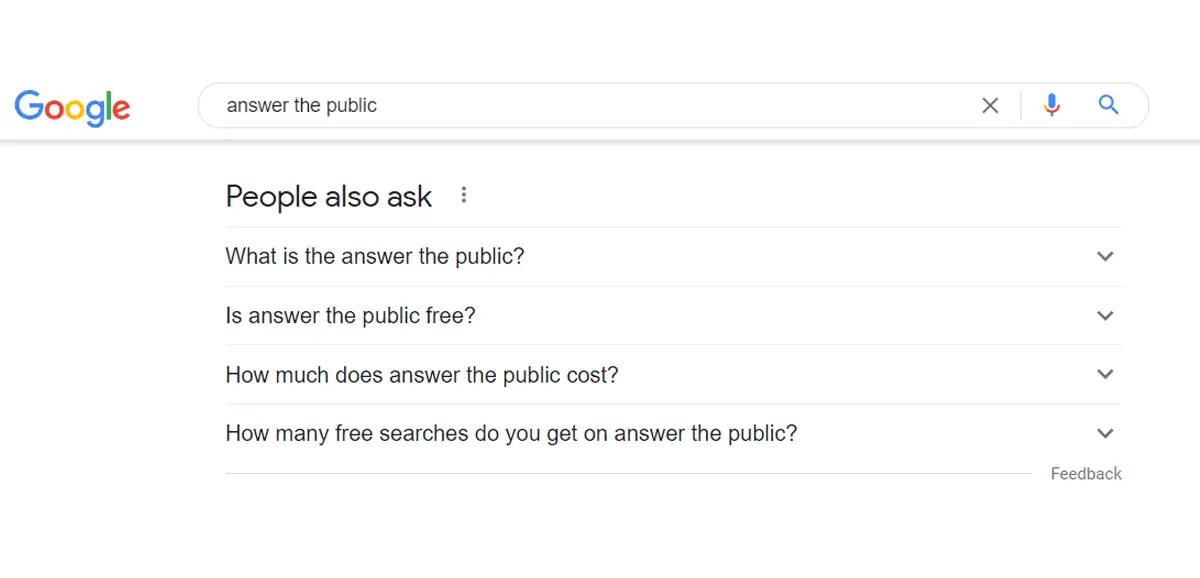A detailed and cleaned-up descriptive caption for the provided image could be:

"A screenshot of Google search results for the query 'Answer the Public.' At the top left of the image is the recognizable Google logo, and to its right is the search input field containing the text 'Answer the Public.' Adjacent to the input field, from left to right, are the icons for 'X' (to clear the search), a microphone (for voice input), and a magnifying glass (to initiate the search). Below this input area is a thin gray separator bar, casting a subtle drop shadow. The main section of the results page shows the heading 'People Also Ask' in large, bold letters. Underneath this heading, there are four related questions: 'What is Answer the Public?', 'Is Answer the Public Free?', 'How Much Does Answer the Public Cost?', and 'How Many Free Searches Do You Get on Answer the Public?'. Each question has a downward-facing drop-down menu arrow on the far right, colored in gray, indicating that more information can be expanded. At the bottom of this section, the word 'Feedback' appears, likely a link for user input on the search results. The background of the page is predominantly white, creating a clean and minimalistic look with minimal distractions. The search input field itself is bordered by a thin, light gray line, and the overall layout emphasizes clarity and user-friendliness."